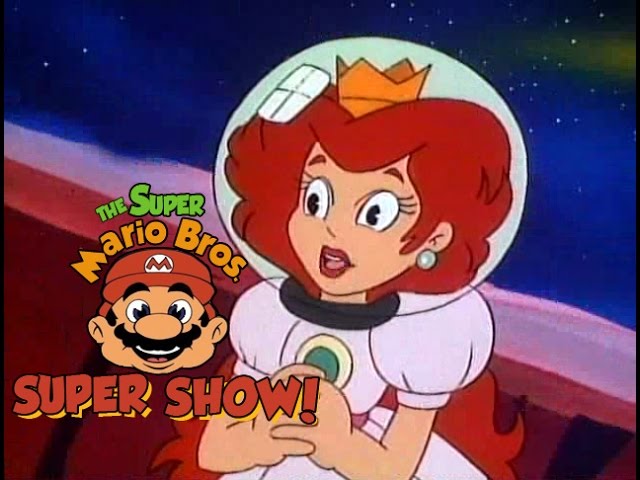This cartoon illustration features Princess Toadstool from the Super Mario Brothers series. She has short, orange-red hair enclosed within a clear space helmet or bubble, complementing her pearl necklace and gold crown. The princess is adorned in a light lavender dress with poofy pink sleeves, exuding a whimsical and regal presence. The backdrop sets her against a dark blue galaxy filled with stars and a striking red landmass. To her left, the text "The Super Mario Brothers Super Show" is prominently displayed alongside a smiling image of Mario, who is wearing his iconic red hat with a white circle and a red "M" in the center. The entire scene captures a blend of outer space adventure and classic Mario charm.